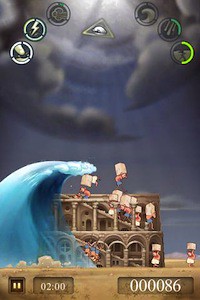The image is a still from a video game. The upper portion of the image features a prominent, though partially cut off, light source at the very top. Radiating beams of light fan downwards, piercing through dark, swirling clouds that create a circular pattern. This circular formation is interrupted at the bottom, revealing a glimpse of the sky.

Within the cloud circle, several icons can be observed. Positioned on the upper quarter of the image, three icons are on the left, one in the center, and another three on the right. The icons on the left have a distinct white outline. The central icon resembles a lightning bolt encased within a white circle, itself set inside a triangle. The icons to the right are also circular, with the bottommost icon featuring a yellow outline, and the one above it to the left having a green outline.

The lower third of the image hosts an intriguing scene: on the left side, a towering wave of water is advancing towards the right side, where a structure resembling a house or possibly the Colosseum stands. Scattered around the structure are multiple characters dressed in red shirts and blue pants, each carrying bricks on their backs, seemingly oblivious to the impending wave.

At the very bottom of the image, the game's interface elements are visible. The bottom left corner displays a pause button. To its right is a clock showing the time as 02:00, and further to the right is the score, which reads 00086, indicating a score of 86.